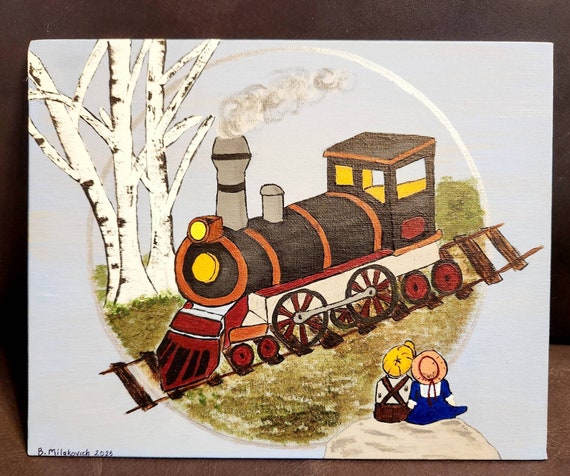This image is a detailed and vibrant drawing by the artist B. Malachowicz, created in 2023, that evokes the charm of a child-friendly scene. The artwork depicts a steam engine train chugging along a track set amidst a grassy landscape, all enclosed within a circular border. The train, predominantly brown with touches of reds, oranges, blacks, and yellows, emits white smoke from its gray steam pipe and features a red front section and both large brown and small red wheels.

In the foreground, two children, a boy and a girl, sit side by side on a cream-colored rock, their backs turned to the viewer as they gaze at the passing train. The boy sports a yellow cap and brown overalls with crisscross suspenders, while the girl dons a pinkish peach hat paired with a royal blue dress. Surrounding them, the scene includes tree branches and lush green grass.

The background is a white canvas, possibly painted with either pencil or paints, placed on a surface that suggests a photograph of the drawing. Shadows cast behind the drawing add to its realistic presentation. This delightful and cozy illustration would make a perfect addition to a child’s room.